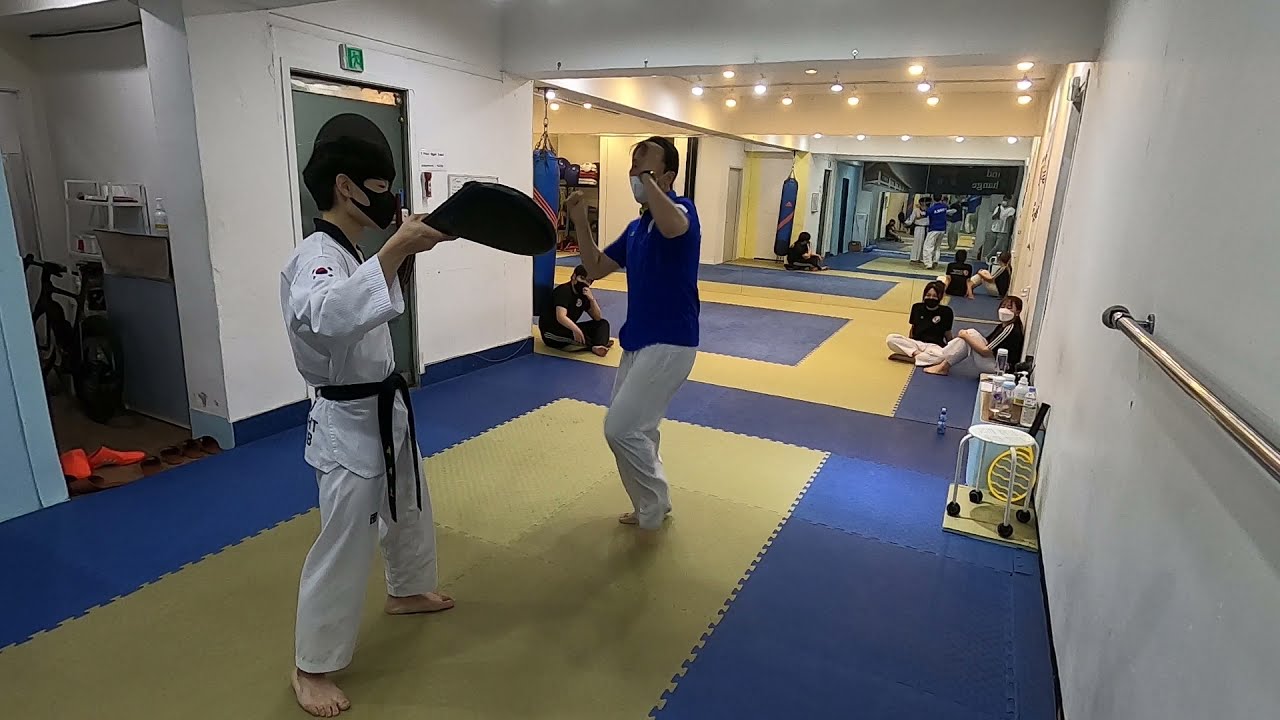In this horizontally aligned rectangular photo, we see a small martial arts dojo with white plaster walls and interlocking blue and yellow puzzle mats covering the floor. The main focus is on two individuals sparring in the center of the dojo. The person on the left, a young man with short black hair, has a black face mask and wears a traditional white martial arts uniform with a black belt. He holds a punching target in his right hand. Opposing him, another man with a white face mask is dressed in white pants and a blue short-sleeve shirt. He has short brown hair that is partially bald on top and might be wearing glasses. 

Behind them, multiple people are seated in a cross-legged position, attentively watching the sparring match. Most of the observers are dressed in black tops and are also wearing face masks, suggesting this was during the COVID-19 pandemic. The dojo features a significant mirror on the far side wall, reflecting the room and its occupants. Additionally, there’s a gray door with an exit sign above it on the left side of the image, and a small adjacent room can be seen behind the young man in white, containing a parked mountain bike.